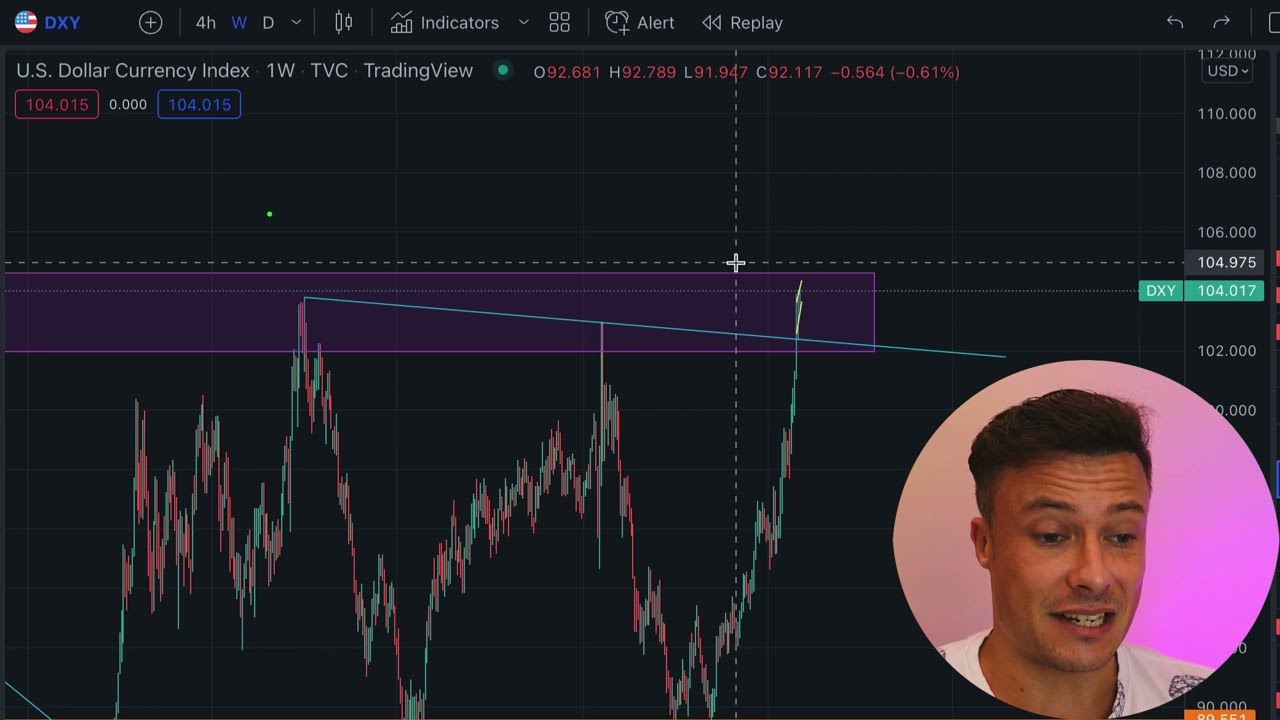The image is a screenshot of a computer screen displaying a graph related to the U.S. Dollar Currency Index. The background of the screen is predominantly black or very dark gray, enhancing the visibility of the graph. The graph features jagged red and green lines indicating fluctuations, along with a horizontal purple bar and a blue line marking the peaks. At the top of the screen, white and red text reads "U.S. Dollar Currency Index" and "1WTVC Trading View," suggesting this relates to financial analysis or trading activity. The y-axis on the right-hand side is labeled with descending numbers, starting from 110 down to 106. In the bottom right corner, there's a small circular image with a pink background. The circle contains a young man with short, dark brown hair and a slightly tanned complexion, wearing a white shirt. He appears to be talking about the graph, likely recording a video or conducting a live stream. The entire composition suggests a detailed financial analysis presentation.